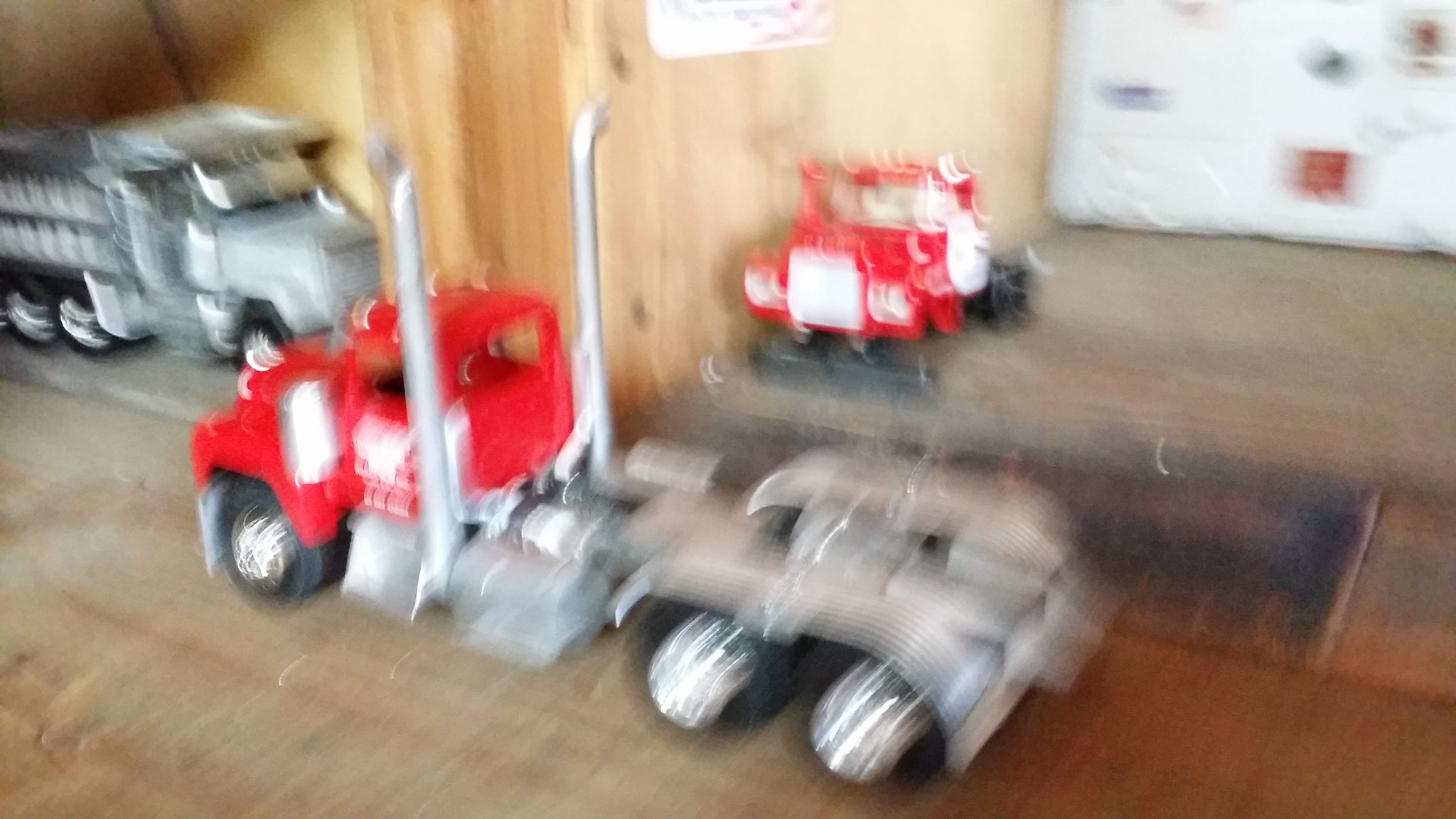The image features a landscape-oriented photograph of three model trucks, displayed on a wooden surface. Central to the image is a red truck with a predominant red body and silver accents, including the base and wheels, suggesting the usual absence of a box attachment on its back. Above this centerpiece, a smaller red truck is visible, appearing diminutive in comparison. On the left side of the frame, an all-gray dump truck completes the trio. The photograph is notably blurry, likely due to camera movement during capture, causing all the vehicles to be out of focus and lacking in discernible details.